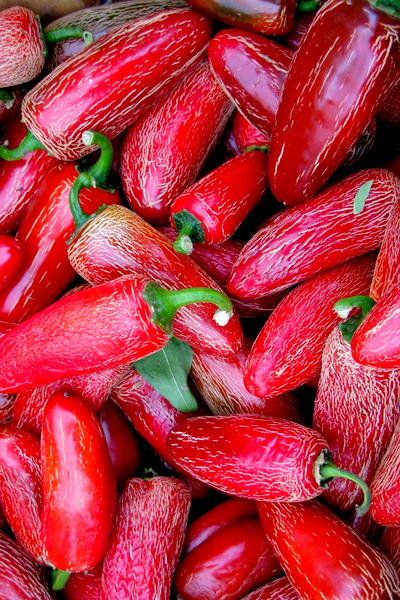This is a vibrant and highly detailed close-up photographic image of red ripened jalapeño peppers. The peppers, in various shades of red, are adorned with a multitude of white lines and markings, giving them a slightly aged appearance. Some are starting to dry out, featuring wrinkles on their otherwise shiny skin. They are arranged haphazardly, overlapping in different directions, with bright green stems that gradually taper off to white tips where they have been cut. In the midst of the peppers lies a single green leaf, adding a touch of contrast. The photograph captures a market-like scene, with the peppers looking freshly picked and tossed into a container or possibly scattered across a surface. This composition features peppers of assorted shapes and sizes, making it rich in texture and color.